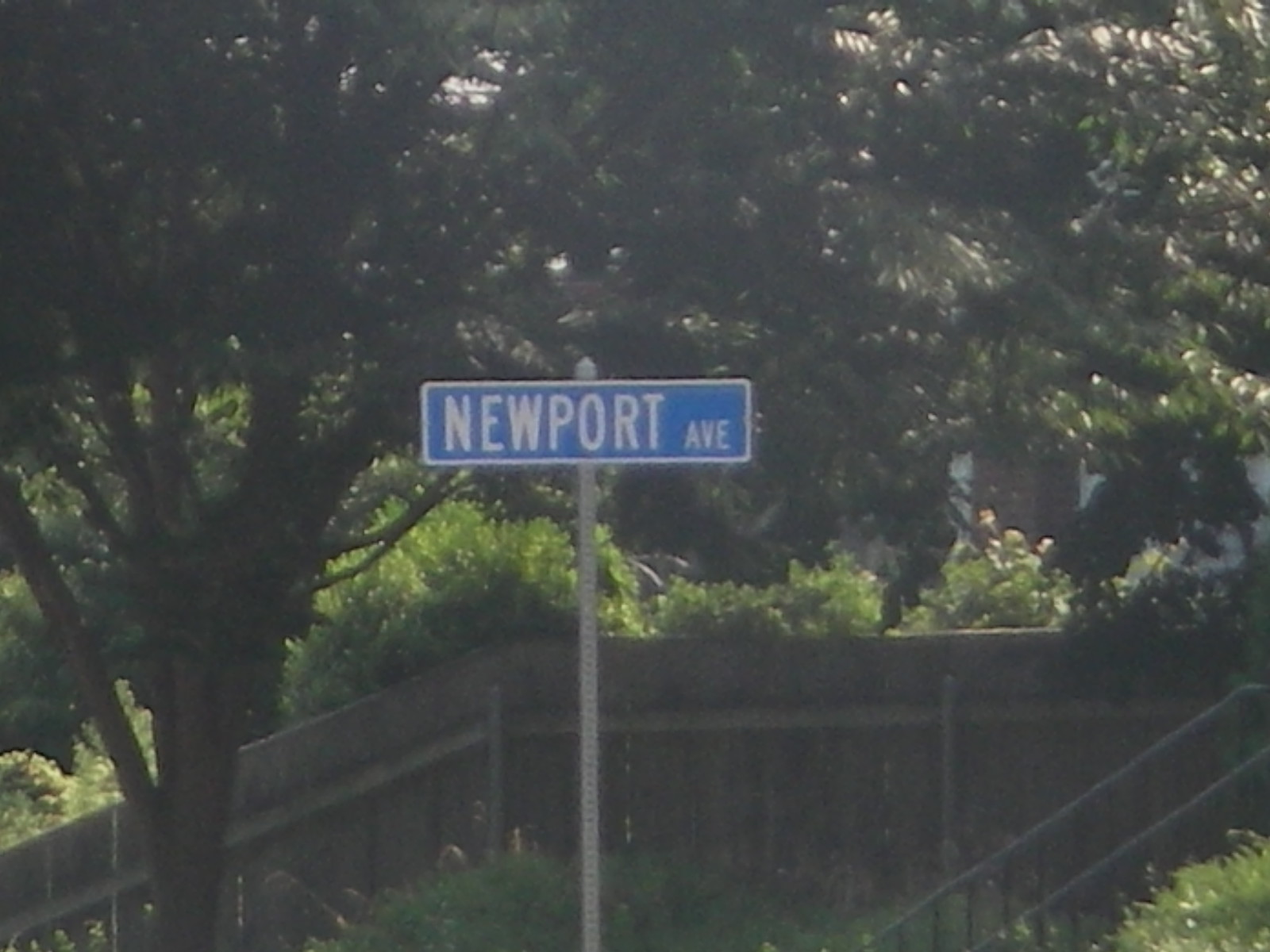This horizontal color photograph captures a street sign in the center of the image, supported by a thin, silver metal post. The sign itself is a blue rectangle with a white border and large uppercase white letters that read "NEWPORT" and smaller uppercase white letters that read "AVE" next to it. The background features a densely packed arrangement of tall trees and bushes with dark green leaves, partially obscuring a brown wooden fence that stretches from the lower left to the middle right of the photo. There are glimpses of a house with a chimney, as well as the banisters of a staircase located in the lower right corner of the image, though the stair steps are not visible. The scene is bathed in daylight but the photo's quality is somewhat blurry, and large tree limbs with thick foliage extend across the upper portion and left edge of the image. The overall composition suggests that the sign overlooks a fenced-in yard.